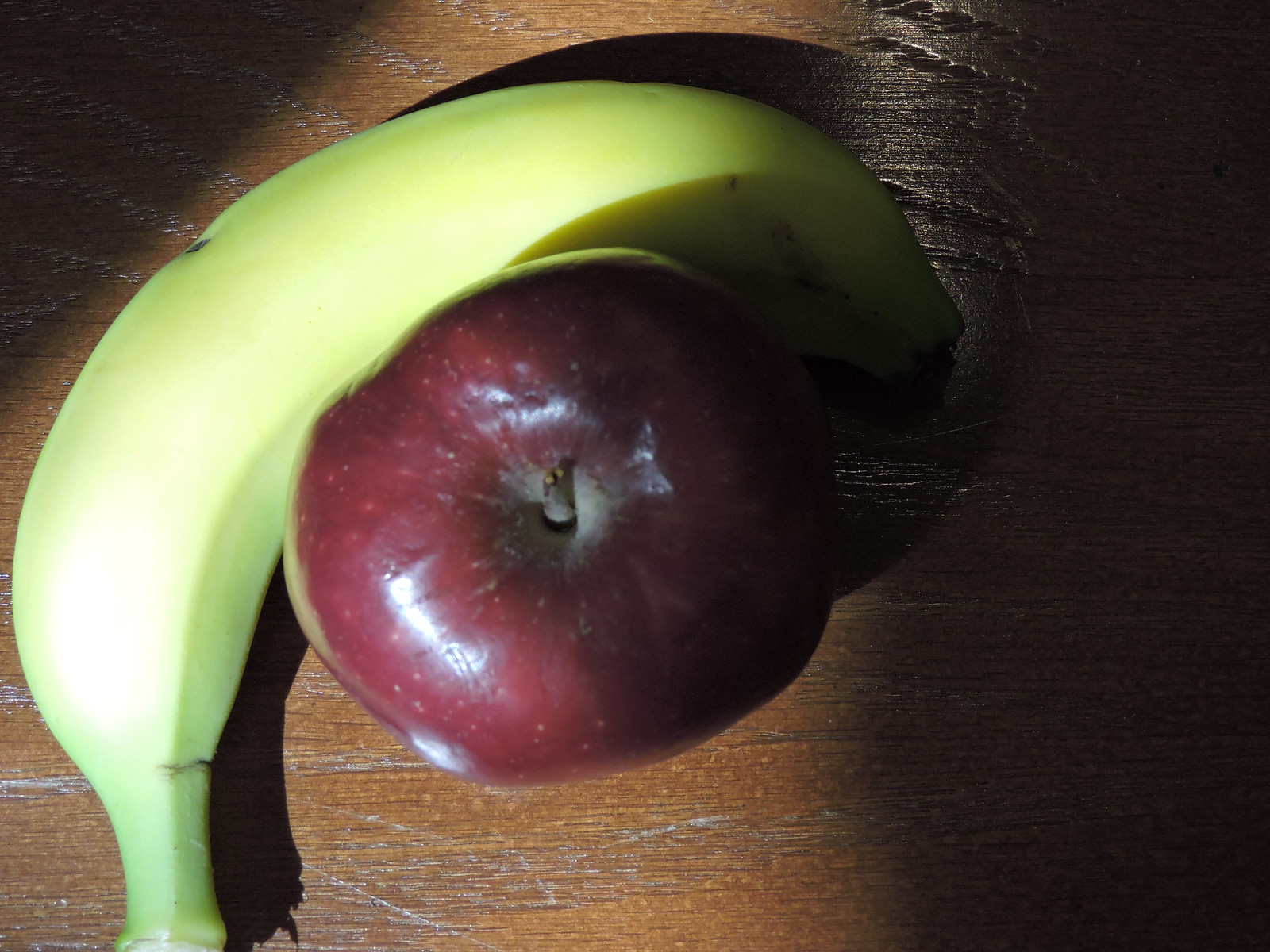In this captivating photograph, a slightly unripe banana lies on its side, gently cradling a moderately smushed apple, creating an almost affectionate scene reminiscent of a cuddle. Both fruits rest on a wooden surface, likely a table, bathed in soft natural light that suggests the presence of a nearby window. The banana, nearing ripeness but not quite there, has a broken stem indicating a premature attempt to open it, yet it remains largely unblemished except for a small indentation on its back. The standing apple, although a bit smushed and imperfect, has a broken-off stem, adding to its rustic charm. Subtle shadows around the fruits enhance the overall composition, making the humble still life both inviting and evocative.